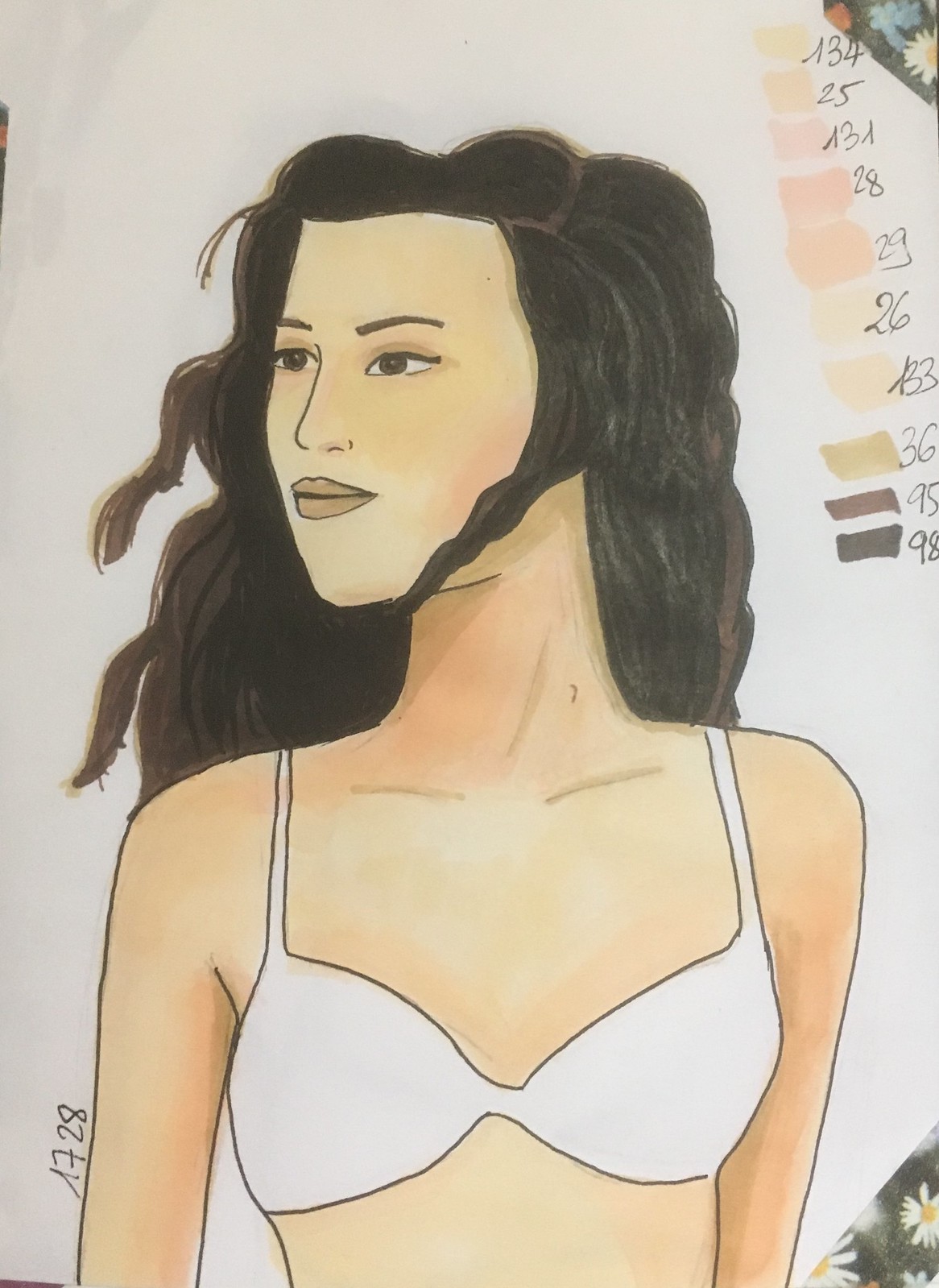This image presents a detailed photograph of a watercolor painting or a meticulously illustrated drawing, possibly created with markers or ink. The artwork portrays a thin woman with long, dark, wavy hair extending past her back, her head slightly turned to her right, revealing more of the left side of her face. She has brown eyes, defined cheekbones, and a prominent clavicle, accentuated by brown eyebrows and subtle eyeliner. Her lips and facial features are finely detailed.

The woman is scantily clad in a simple white bra, contributing to a minimalistic aesthetic. On the right side of the artwork, there is a sequence of color swatches varying from light nude to dark brown, each meticulously labeled with alphanumeric codes such as A34, 25, A3A, A28, A29, A26, A33, A36, A95, and A98. These swatches appear to function as a color reference for the artist.

The artwork is bordered by small, intricate patterns of white daisies on a green background, visible in some corners. Additionally, the number 1728 is marked in brown ink near the woman's arm, adding another layer of detail to the piece. The entire composition appears to be rendered on white paper, enhancing the vividness of the colors and the distinctness of the outlines in black ink.